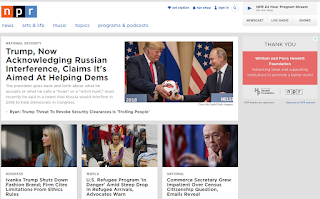Certainly! Here's a more detailed and cleaned-up descriptive caption:

---

This is a small screenshot captured from the NPR news website. The image is enclosed within a dark gray border, framing a large, white rectangular area. Within this white area, there is a smaller rectangle divided into three colored squares, each containing a letter of the NPR logo.

- The first square is orange with a bold, white lowercase 'n'.
- The second square is dark blue with a bold, white lowercase 'p'.
- The third square is cyan blue with a bold, white lowercase 'r'.

To the right of these squares, there is a section where the 'Sign In' button and other navigational buttons are located, although they appear too blurry to read. Adjacent to the 'Sign In' button is a small magnifying glass icon, indicating the search function.

Further to the right, there's a gray rectangle containing a blue play button facing right, which is presumably for listening to audio content, though it's too blurry to confirm.

Below that, there are several gray rectangles:
- The first rectangle prominently displays the word 'Newscast' in black centered text.
- Accompanying this is a partially visible string of text starting with 'L-I-M-I...'

Moving down on the right-hand side, an advertisement appears within a dark gray bezel. The text on it is mostly black, reading 'Thank you,' followed by some red text attempting to deliver a warning, which is too blurred to decipher.

On the left side of the white area, there are several images and captions:
1. A photo of Trump handing an orange and red soccer ball to Putin. Above, the headline reads in bold black text: "Trump now acknowledges Russia's interference, claims it's aimed at helping Dems."
2. Below, an image of Ivanka Trump in a blue dress and with shoulder-length blonde hair. The distorted text partially reads: "Ivanka Trump, [shorts/crown/fashion], B-R-E-N-E-L, F-L-I-N-N, cities... provide..."
3. Continuing downwards, an image of a little girl wearing a tan vest and purple shirt, standing amongst other individuals, with a child in gray behind her. The caption beneath indicates: "U.S. refugee program in danger..." though the rest is blurred.
4. Further down is a photograph of an older Chinese man wearing glasses, next to an American flag, and the obscured text mentions a commerce secretary and someone named Martin.

The combination of these elements captures a snapshot of the diverse news coverage and user interface features on the NPR website at that moment.